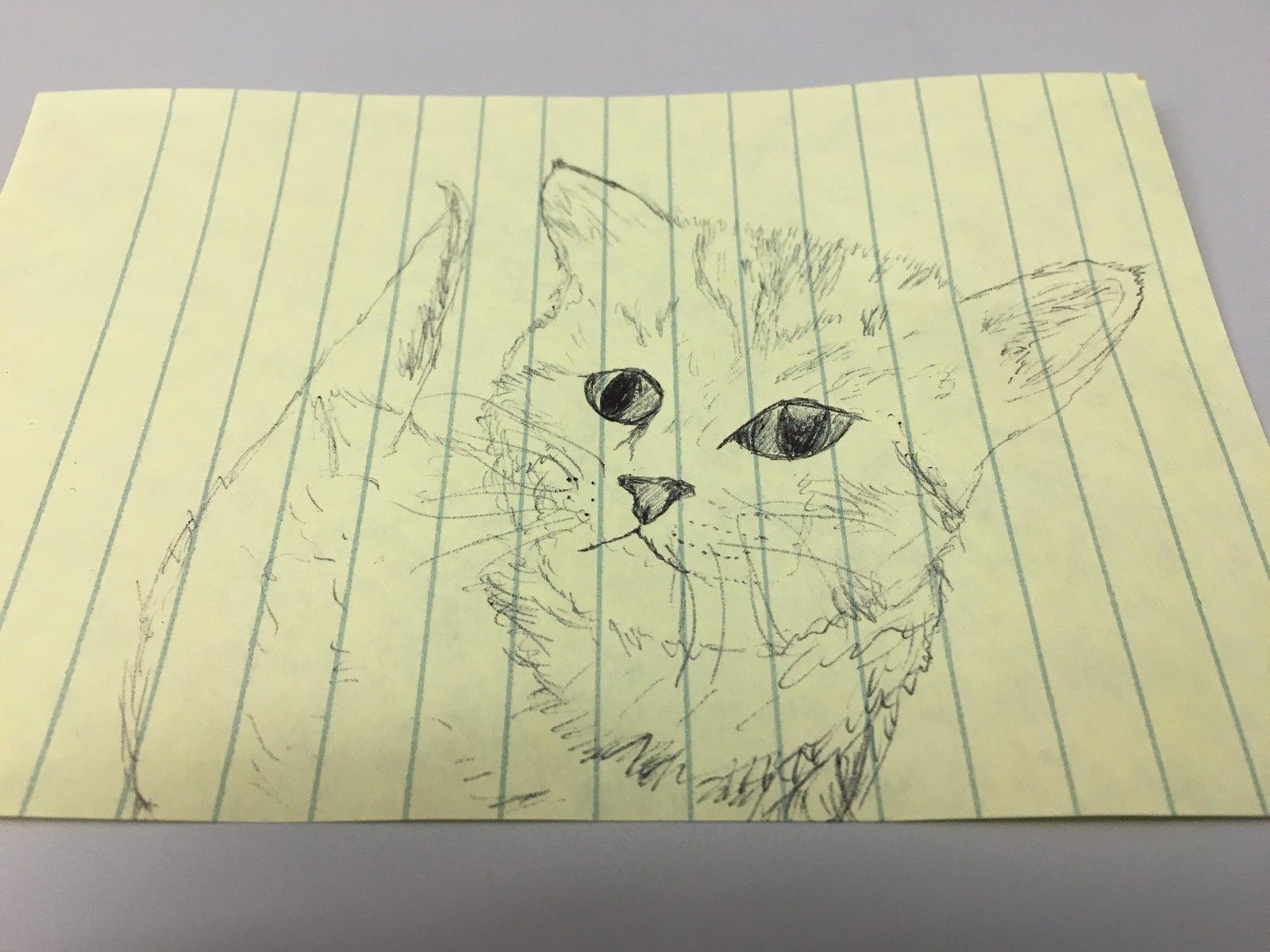A highly detailed drawing of a cat is rendered on yellow paper adorned with blue stripes, reminiscent of legal pad paper. The artist, showcasing evident talent, has skillfully captured the cat’s distinct features: its fur is meticulously detailed, eyes are expressively drawn, and whiskers are clearly defined. The texture suggests the use of a pen, likely black though not definitively. The cat’s ears add character to the drawing; the left ear appears slightly floppy, while the right ear stands more alert and perked up.